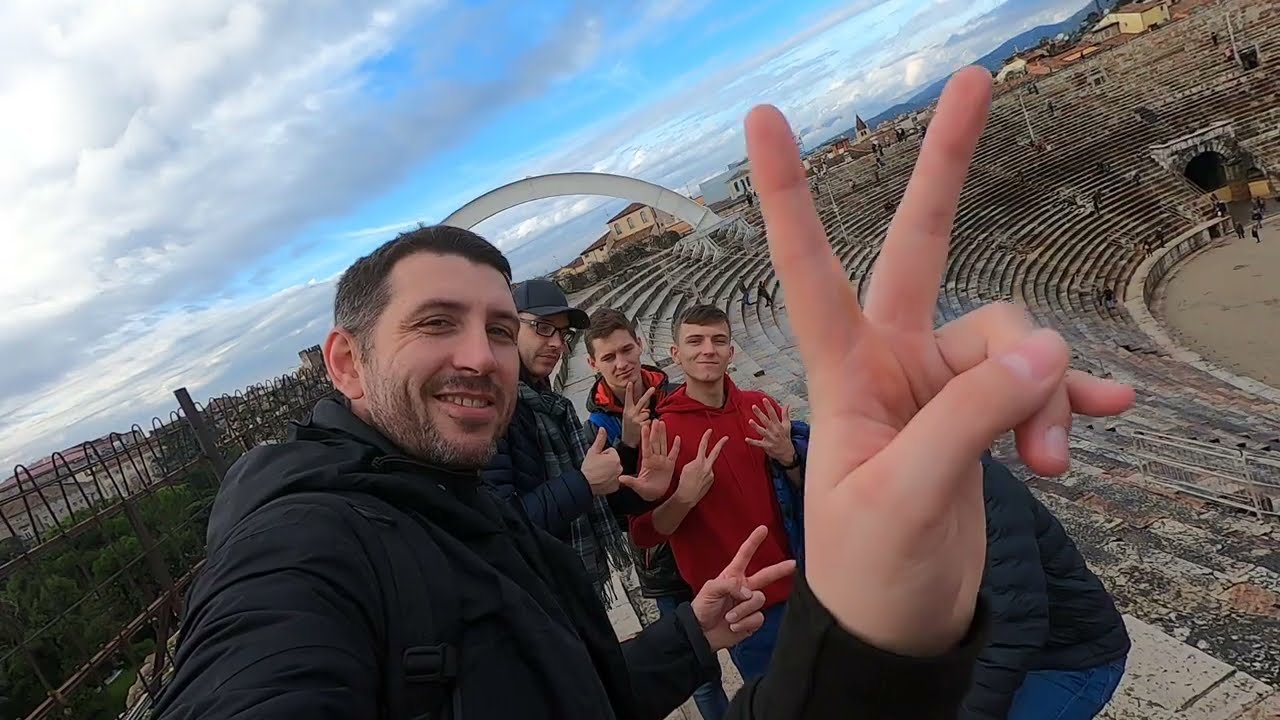In this outdoor scene set against the backdrop of an ancient amphitheater with many tiers of stone seating, four men are capturing a selfie on what appears to be a slightly chilly, partly cloudy day with a blue sky dotted by white clouds. The men are positioned on stone steps, likely vacationing or sightseeing. The man closest to the camera is wearing a dark jacket and smiling, while holding up a V sign with his fingers. Beside him, a middle-aged man, also in a dark jacket, sports glasses and a black baseball cap, giving a thumbs up with one hand and holding the other hand up, showing all his fingers. In the background, two younger men are mimicking the hand gestures, with one raising a peace sign and the other showing all his fingers. Beyond the ancient structure, some distant buildings or housing are visible. An additional hand with a peace sign is seen in front of the camera, likely belonging to someone just outside the frame. The amphitheater's historic, weathered stonework frames the cheerful group's smiles, hinting at a memorable and joyous moment.